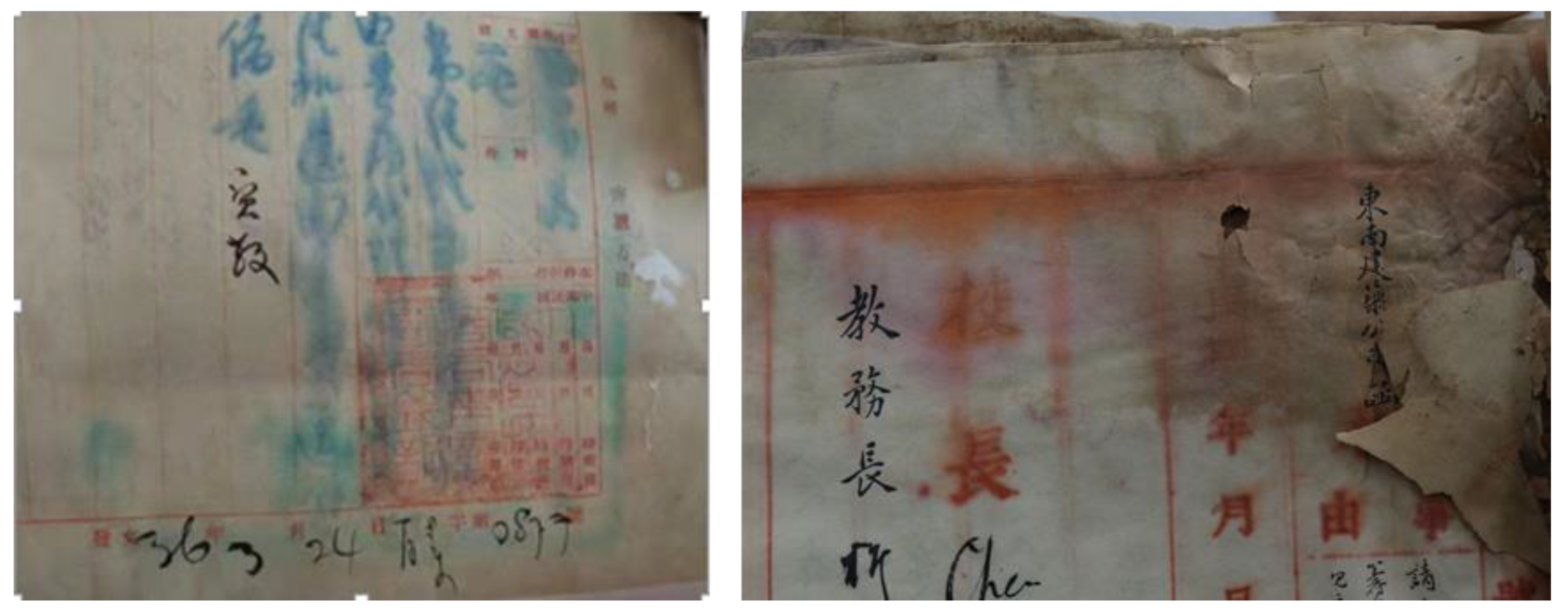In this image, there are two side-by-side photographs of what appear to be aged and worn pieces of paper bearing Japanese characters. Both pieces of paper are brown, with frayed and shredded edges that suggest their old and rough condition. The paper on the left features multiple rows of characters written primarily in blue ink, with a few black characters interspersed. The blue ink is smeared, as if the paper had been wet, and at the bottom of this piece, numbers "3624" are discernible. Overlaying the blue characters is a red stamp, adding another layer of red characters. The right photograph seems to be a close-up of the red-stamped area from the left paper. It shows a row of black characters, followed by two smeared red characters with a black one underneath. The ink on this portion is notably smeared and runny, which further accentuates the aged and damaged nature of the document.